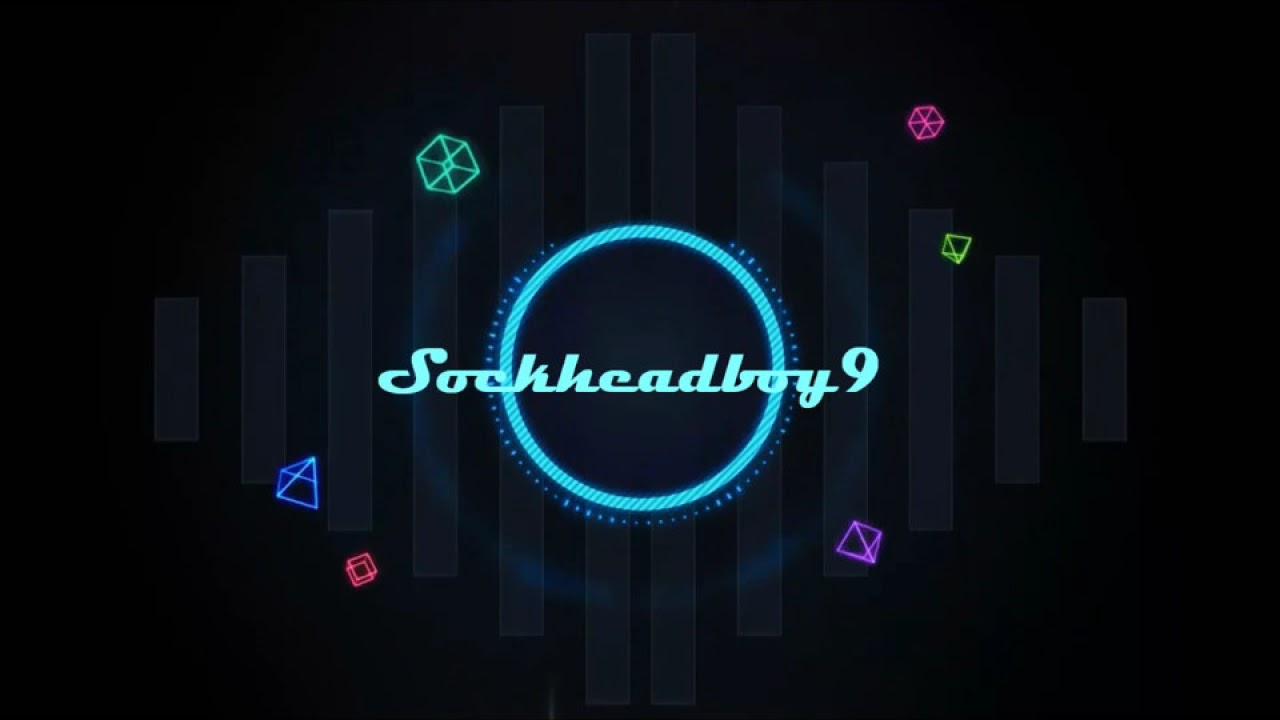This digital artwork or logo features a striking design centered on a neon light blue circle with a navy blue interior. The circle's outline is adorned with numerous neon blue polka dots, though the top section is missing some dots. Overlapping the circle is the cursive text "Sock Head Boy 9" in seafoam green font. The background is entirely black and is interspersed with very dark gray vertical bars; these bars are tallest in the middle of the image and gradually decrease in height towards the edges. Additionally, floating around the circle are various geometric neon 3D shapes, including cubes, triangles, and squares, in colors such as aqua, blue, red, purple, and green, all drawn with glowing lines, adding a sense of three-dimensionality and vibrancy to the composition.